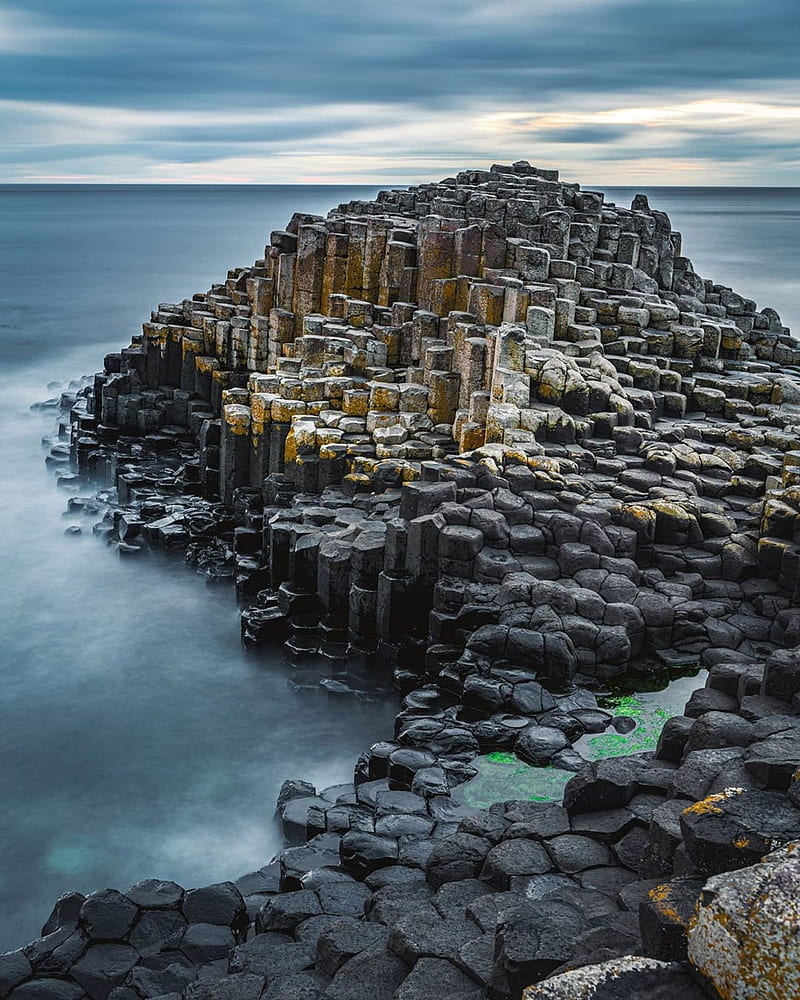The image captures the iconic Giant's Causeway, a renowned natural stone formation on the coast of Northern Ireland. This remarkable geological structure is composed of hundreds of vertically jutting, thick, angular stones that appear to form stepped, uneven columns of varying heights. These basalt columns create a striking visual effect, transitioning in color from light gray in the center to yellowing stones and further to charcoal-colored rocks towards the foreground. The stones are interspersed with pools of water, some hosting vibrant green algae. The scene is set against an overcast sky, imparting a gloomy, almost mystical atmosphere, with dark, cloudy skies and a gray sea surrounding the formation. The coastline and ocean water appear dark blue, adding to the dramatic ambiance of this ancient volcanic landscape. No text or other objects are present in the picture, allowing the raw beauty of the Giant's Causeway to stand in stark prominence.